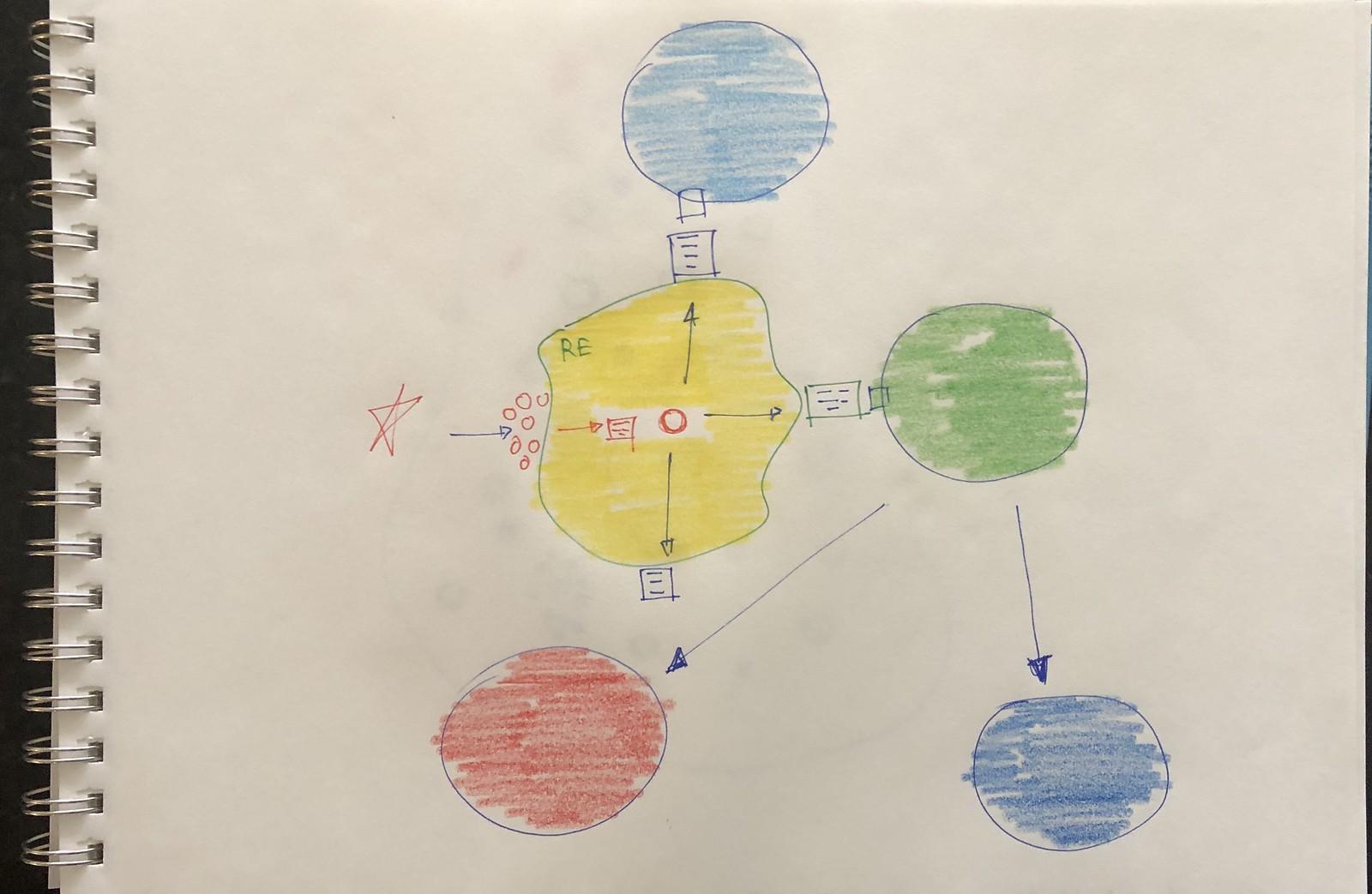This photograph captures a detailed drawing on a spiral-bound drawing pad, with the pad’s spirals positioned slightly right of the left edge of the image. The hand-drawn masterpiece features a variety of shapes and colors that are meticulously arranged on a white background.

Prominently in the upper section of the drawing, there is a blue circle with a smaller square positioned at its bottom. Directly beneath this is a yellow, irregularly shaped blob. To the right of the yellow blob, a green circle is placed, connected by two blue arrows leading to another blue circle located in the bottom right corner of the image. Below and slightly left of the yellow shape lies a red circle.

To the left of the yellow blob, a red star is drawn, accompanied by a small black arrow and a series of tiny red circles that extend from the red star towards the yellow blob. Inside the yellow shape, at its very center, a red circle is encompassed by a small red box and a red arrow stretching from the right to the left.

In the upper left-hand corner of the yellow blob, the letters “R” and “E” are clearly written. Surrounding the blue, green, and red circles, there are three arrows pointing in different directions – upwards, downwards, and to the right, respectively. Between the yellow blob and each of the colored circles and arrows, there are small blue squares with horizontal lines, adding another layer of complexity to the drawing.

This artistic creation is a fascinating interplay of colors, shapes, and directional arrows, captivating the observer with its intricate details and structured layout.